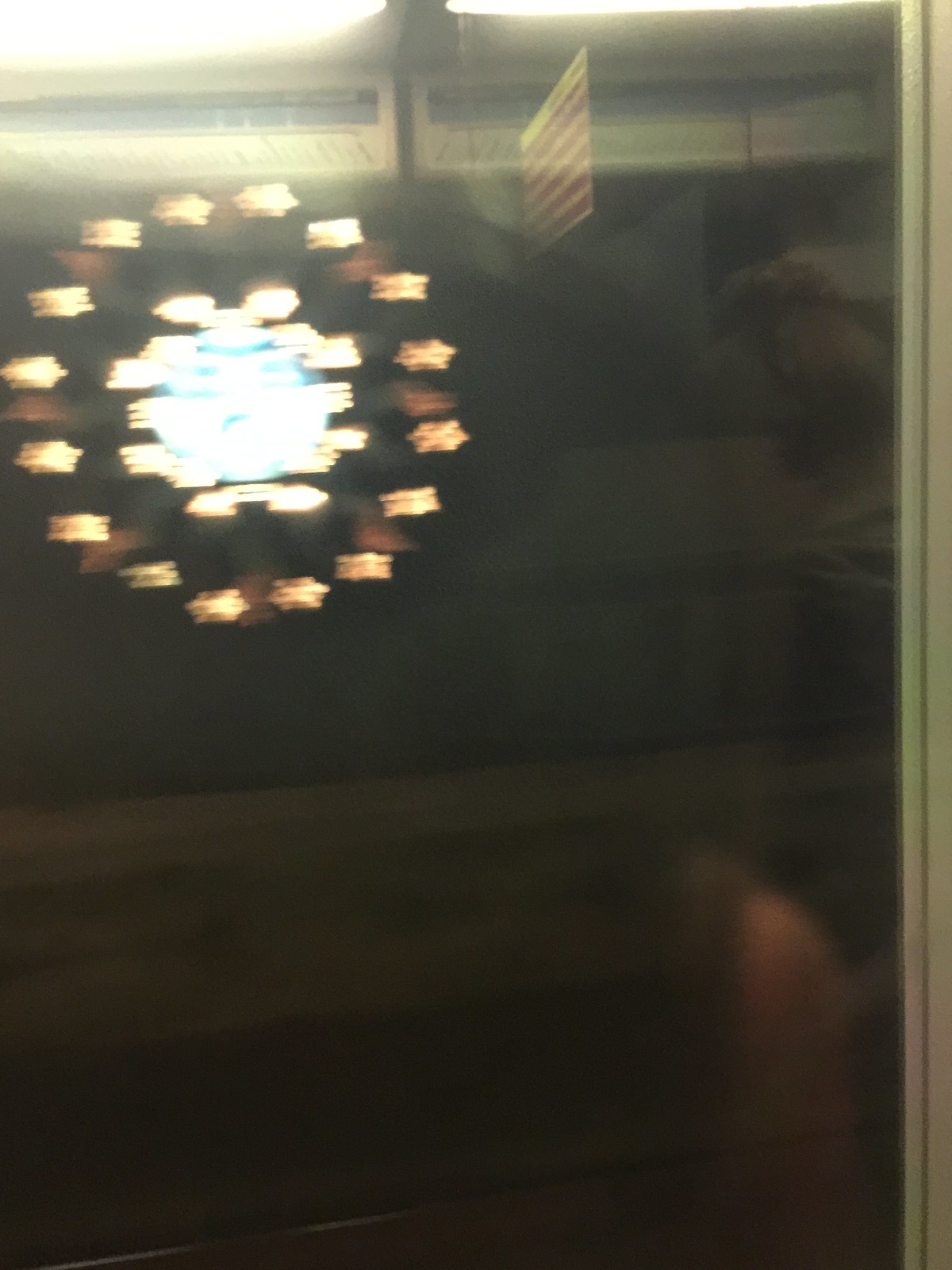This image shows a nighttime scene captured through a window, possibly of a train or a house, with multiple layers of reflection adding to its complexity. The primary focus of the image appears to be a display of fireworks or bright lights in the sky. Central to the image is a large blue circle, radiating bright white lights from its core, surrounded by two expansive rings of yellow stars. The reflection on the glass adds a layered effect, revealing faint images of people, storage areas, a map that potentially resembles a tube station, and a red sign or billboard in the background. The top left corner features a somewhat blurred cluster of circular lights with yellow and brownish hues, reminiscent of a carousel. Additionally, a blue stripe with white accents is visible, though its specific nature remains indistinct due to the blurriness of the image.